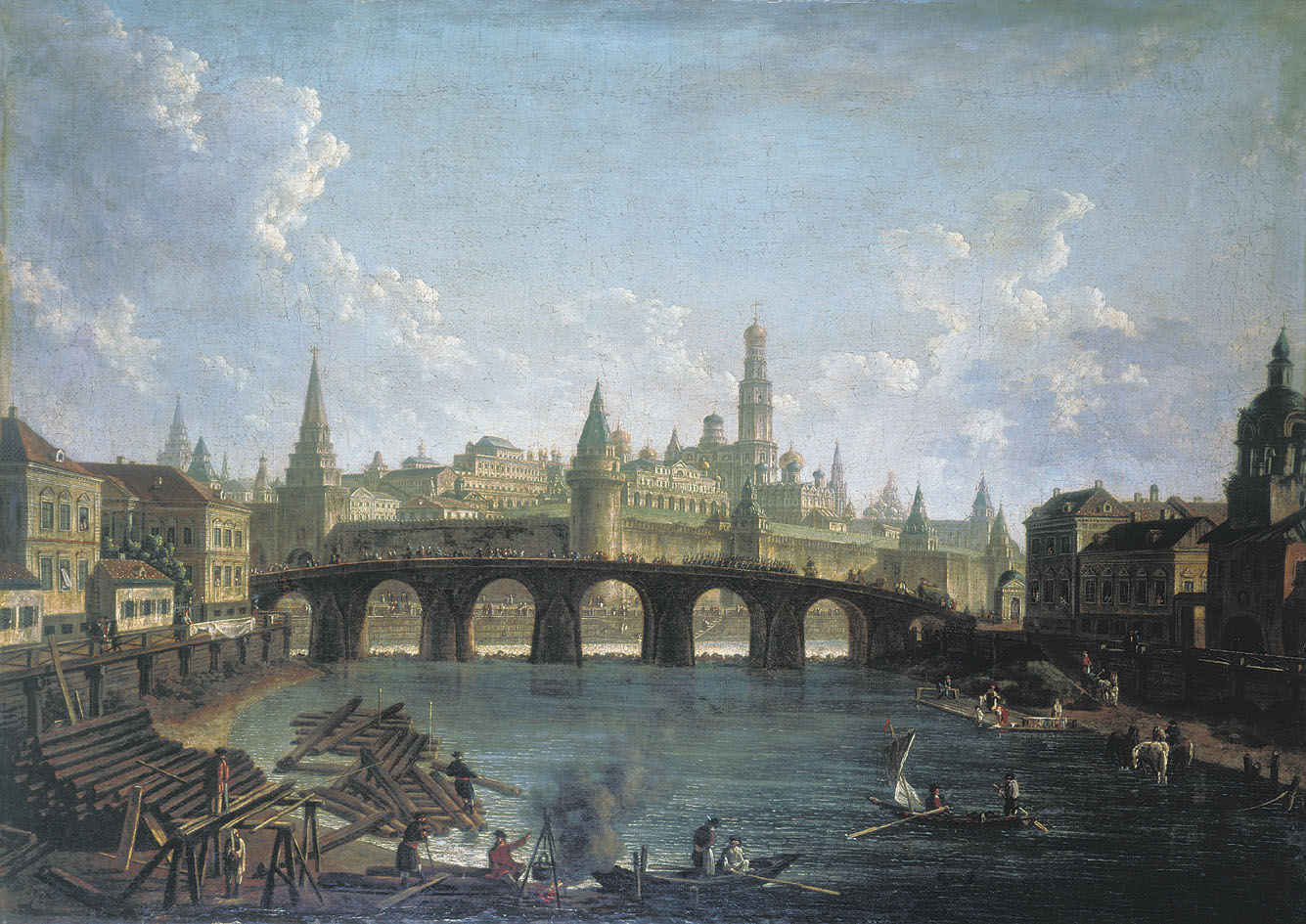The painting depicts an intricate scene of a medieval town with a prominent bridge arching over a serene river. The background reveals a majestic, sprawling cityscape framed by large stone walls and crowned with towering buildings and a notable structure adorned with a shining spire piercing the sky. The sky above is a blend of blue, dark blue, gray, and white clouds, casting a dynamic ambiance over the landscape. 

In the foreground, logs are piled along the left bank, some extending into the water where a figure stands, and a small wood fire with a cauldron suspended by poles burns nearby. The river is animated by several canoes and small passenger boats navigated by people, creating a lively setting. On the right side, a short pier allows others to gaze out over the river’s expanse. Additionally, a horse can be seen in the distance, further enriching the historical atmosphere of the scene. The detailed architectural elements and the daily activities captured in the painting offer a vivid snapshot of a bustling medieval life.